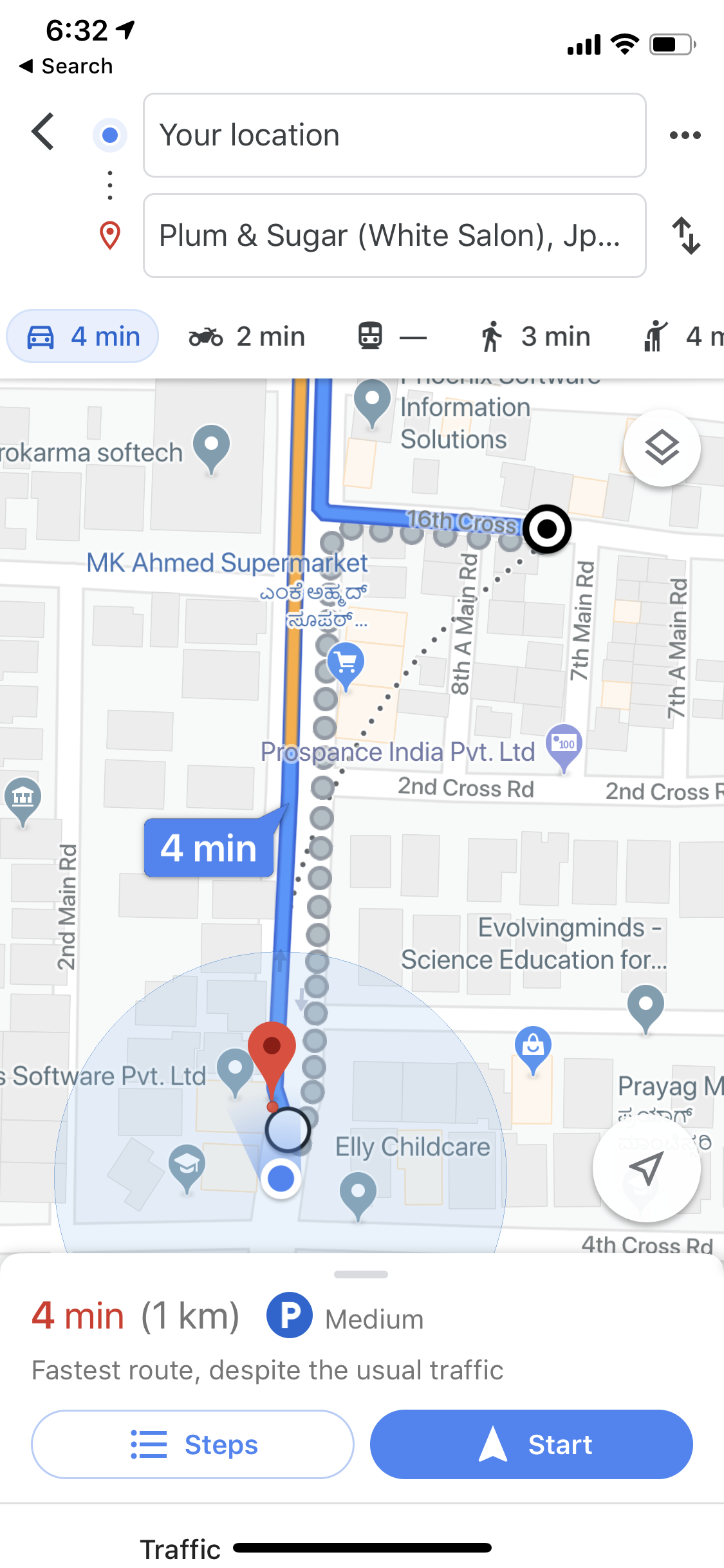This detailed screenshot captures a road map with a vertical road running through its center. The road is distinctly color-coded: orange in the upper half and blue in the lower half. In the upper left corner of the map, against a primarily gray and white backdrop, the business name "SoftTech" is prominently displayed. Directly beneath it, in blue text, is "M. K. Ahmed Supermarket." Shifting to the upper right corner, the map shows more business names, starting with "Information Solutions," followed by "Prosspans India Limited," and "Evolving Minds Science Education." At the top of the map, various transportation icons are shown in light blue boxes, each indicating travel time: a car icon with "4 minutes," a motorcycle icon with "2 minutes," a walking person icon with "3 minutes," and a rider icon also with "4 minutes."